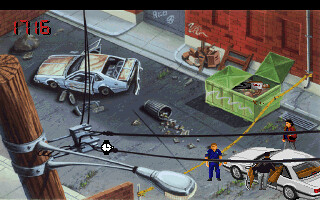This photograph is a low-resolution screenshot of a video game, showcasing a detailed, overhead crime scene set in an urban environment. The scene is depicted with a leaning toward realistic graphics. The road, positioned diagonally from the top left to the bottom right, features two white cars prominently. The first white car, in the middle of the street, appears wrecked with visible rust and damage. A knocked-over trash can spills garbage onto the street beside it, while a large green industrial dumpster with its top open reveals more trash behind. 

In the lower right corner, a second white car is parked with its driver's door ajar, and someone is seen exiting it. A policeman is standing in front of this car, facing the viewer. Three individuals are around the scene: one in a red jacket, another dressed in black and grey seemingly getting into the second car, and a third person near the second car. 

Additionally, part of a streetlight and phone wires are visible in the upper left corner. The upper right section of the image features a red building across the sidewalk. The red digital number "1716" is displayed in the corner of the image, adding to the game-like ambiance. Notably, the foreground includes a small black watch showing the time as 3 o'clock, contributing to the detailed mise-en-scène of this urban crime depiction.